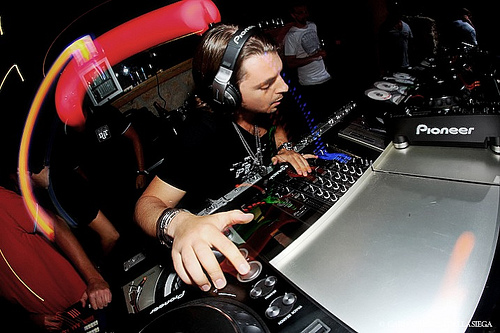The image captures a DJ, a white male with long dark brown, mid-length hair, centered at his DJ sound equipment. He is wearing a black T-shirt with a white pattern on the front and a long necklace around his neck. His gaze is directed downwards as he intently manipulates the numerous knobs, buttons, and switches of his Pioneer-branded equipment. He is adorned with black Pioneer headphones. The scene features a palette of black, white, gray, silver, red, orange, yellow, peach, and electric blue, with a touch of maroon. Behind him, the background is dimly lit and blurred, with indistinct figures, including one person in a white T-shirt. To his left, only an arm and torso of another man are visible. The setting suggests he is performing in a club, and the proximity of the shot implies it might have been taken by a professional photographer.